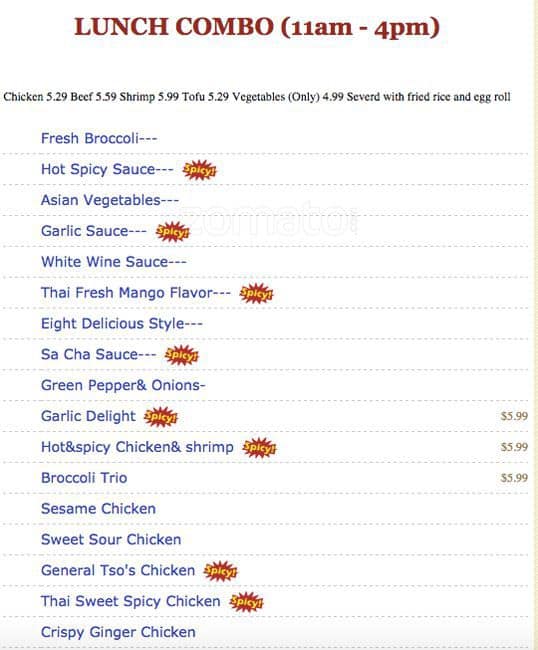**Lunch Combo Menu**

**LUNCH COMBO** (11am-4pm)

---

This menu portrays a simplistic yet enticing layout ideal for lunchtime. The title "LUNCH COMBO" is prominently displayed at the top in bold, all-capital, maroonish-red letters, perfectly centered with the time frame (11am-4pm) in parentheses beneath it. The clean design includes a noticeable white space beneath the title, juxtaposed with a single yellow border running down the right side, subtly guiding the eye.

Under this white space, the pricing for protein choices is clearly listed:
- Chicken: $5.29
- Beef: $5.59
- Shrimp, Tofu, and Vegetables: $4.99 each

Accompanying each combo, the menu offers syrup with rice and an egg roll, ensuring a complete meal.

**Selections:**
- Fresh Broccoli
- Hot Spicy Sauce
- Asian Vegetables
- Garlic Sauce
- White Wine Sauce
- Thai Fresh Mango Flavor
- Sacha Sauce (delicious style)
- Green Pepper and Onions
- Garlic Delight
- Hot and Spicy Chicken and Shrimp
- Broccoli Trio
- Sesame Chicken
- Sweet and Sour Chicken
- General Tso's Chicken
- Sweet and Spicy Chicken
- Crispy Ginger Chicken

Each dish that is specified as spicy is appropriately marked with a "spicy" icon, ensuring customer awareness. Additionally, three popular selections have prices clearly indicated next to them:  
- $5.99

This detailed and carefully structured menu ensures clarity and appeal, making it easy for customers to decide on their lunch choice.